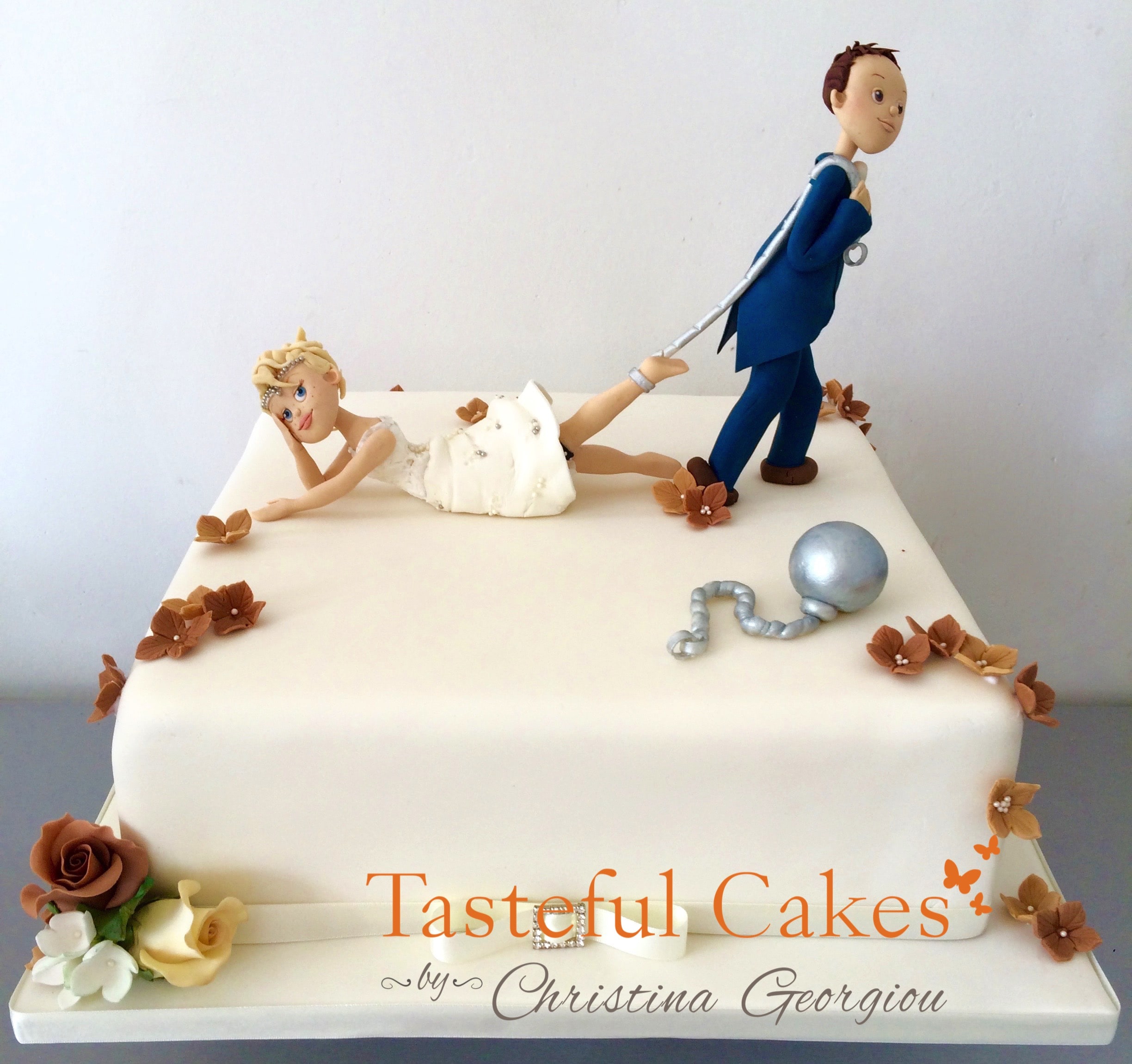This photograph showcases a square wedding cake featured in an advertisement for Tasteful Cakes by Christina Giorgio. The cake is elegantly adorned with creamy white fondant frosting and is decorated with fondant flowers. On the bottom left corner, there are larger fondant roses in shades of brown and cream, accompanied by small white flowers. Additional brown flowers ascend from the bottom right corner, spilling over the edge onto the platform. The top of the cake features a playful bride-and-groom figurine scene: the groom, dressed in a blue suit with a rope over his shoulder, pulls the bride by a shackle around her ankle. The bride, with blonde hair, wears a white dress and a tiara and lies on the ground with her hand on her cheek. A ball and chain, unattached, sits on the bottom right corner of the cake. The display is set on a gray platform with a white background. Text at the bottom of the image reads "Tasteful Cakes" in orange with accompanying butterflies, and below it, "By Christina Giorgio" is written in elegant cursive.